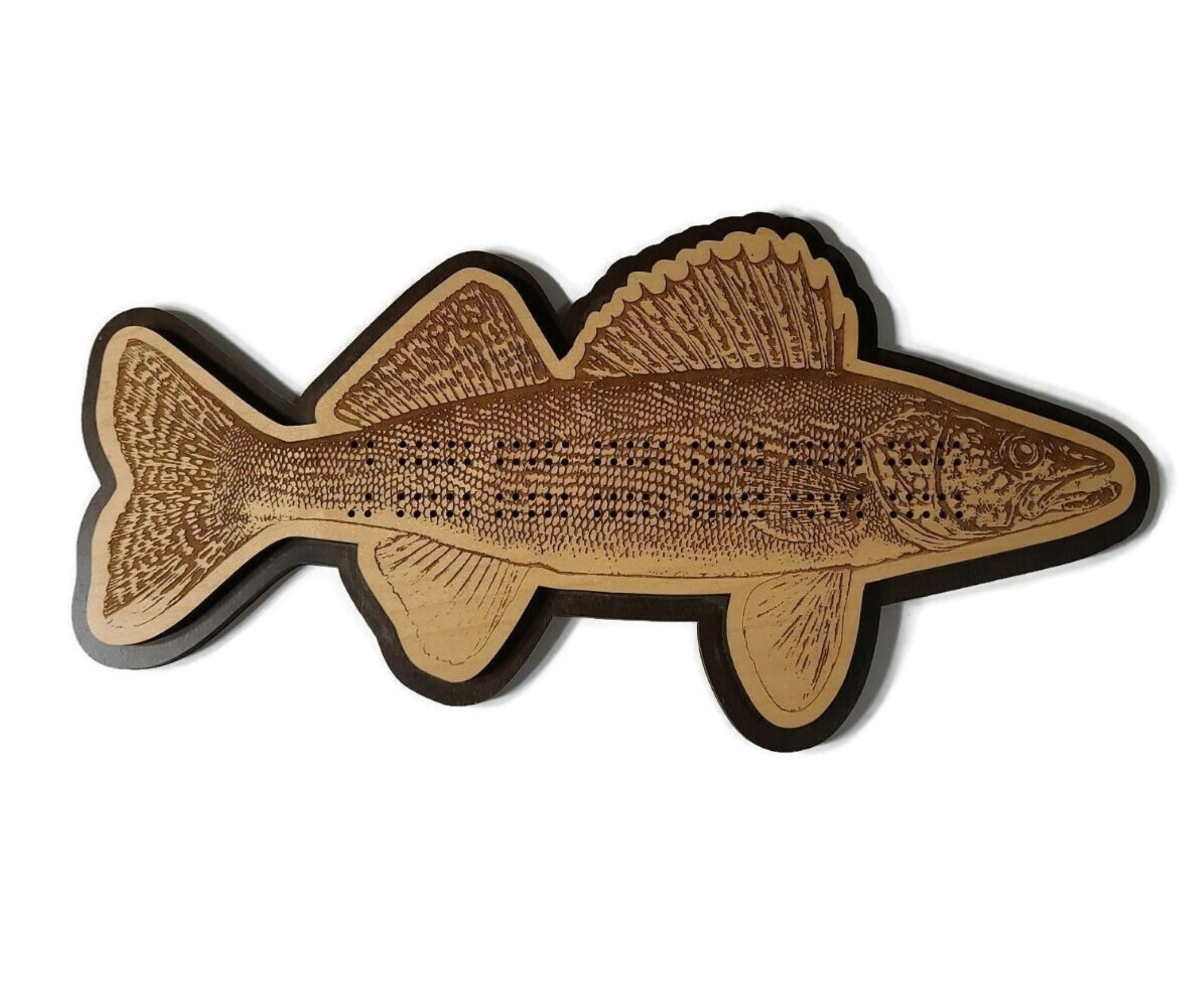This image showcases a meticulously crafted decorative fish, likely intended as a unique wall-mounted piece for home decor. The fish appears to be sculpted from wood and painted in shades of reddish-brown, featuring intricate detailing to mimic a real trout. The body of the fish is adorned with painted scales and a clearly defined face with an open mouth. It has five fins in total: one prominently serrated and jagged fin on the back, with four smoother, lighter-colored fins positioned on the body. The surface is speckled and includes several pegboard-like holes arranged in two rows starting from the gills and extending nearly to the tail. The entire fish is bordered by a black or dark brown outline, enhancing its three-dimensional look. The overall appearance suggests a combination of artistic and natural elements, creating a visually striking and detailed depiction that is both rustic and elegant.